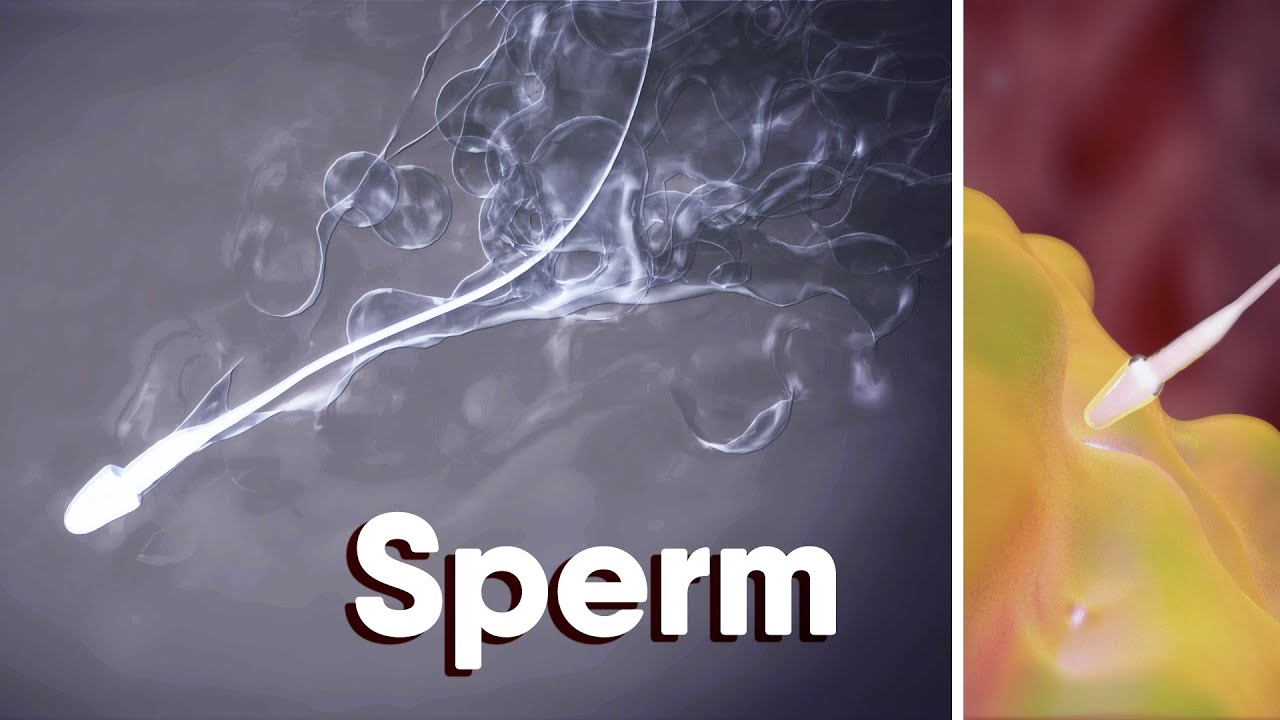This informational digital graphic consists of two juxtaposed images, with the left image larger than the right. The dominant left section showcases a white sperm with a singular, squiggly tail, set against a grayish-blue background. This image also includes white, large thick letters outlined in black that spell "Sperm." The smaller right-hand image transitions to a scene where the white head of the sperm is closely approaching a textured yellow surface, representing an egg, against a red background. This composite illustration effectively demonstrates the process of sperm attempting to fertilize an egg.